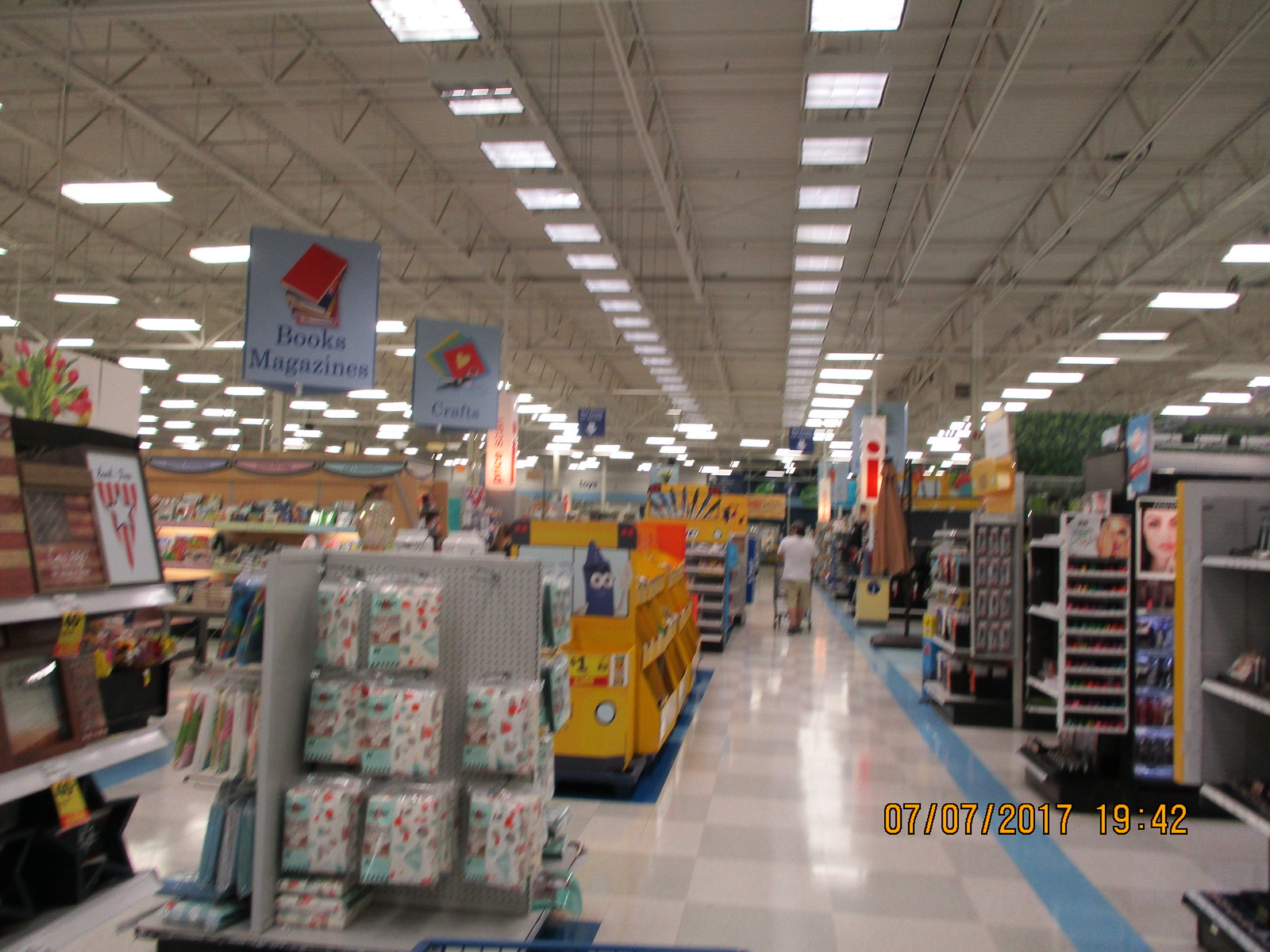The image depicts a long aisle within a large department store, characterized by a white and gray checkerboard patterned tile floor with a blue line spanning its length. Overhead, the white ceiling has exposed beams and multiple rows of square fluorescent light fixtures. The aisle is populated with several displays. On the left, there is a small display for party tablecloths and, behind it, a corner shelf showcasing framed prints. Centrally, a prominent yellow cardboard bus-shaped Crayola display is filled with markers and crayons in various pockets. On the right, a nail polish display is adorned with signs showing women applying nail polish. Further down the aisle, a person in a white t-shirt and tan shorts (or hockey pants, according to one description) is seen pushing a cart. The bottom right corner of the image bears a timestamp reading 07-07-2017 and 19:42.